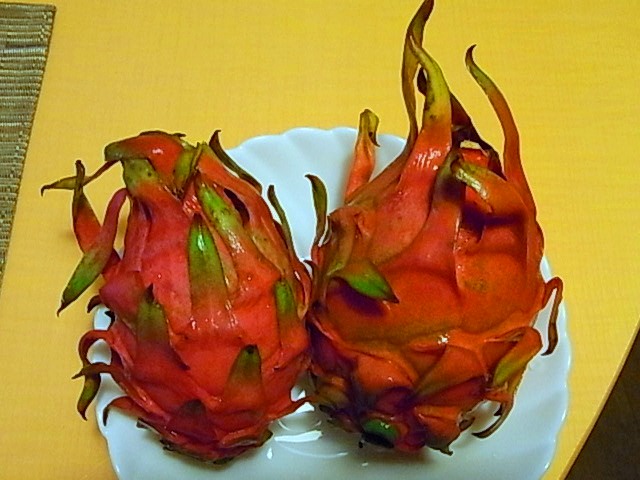In the photograph, two dragon fruits are prominently displayed on a white plate, which rests on a vibrant yellow surface, possibly a table or mat. The striking dragon fruits are bright red with green, leaf-like extensions that give them the appearance of small, flaming balls, reminiscent of pineapples with fiery flares. This vivid ensemble creates a captivating focal point against the white plate and yellow background. Additionally, a portion of a cloth is visible on the left side of the image, subtly enhancing the composition's texture and depth.